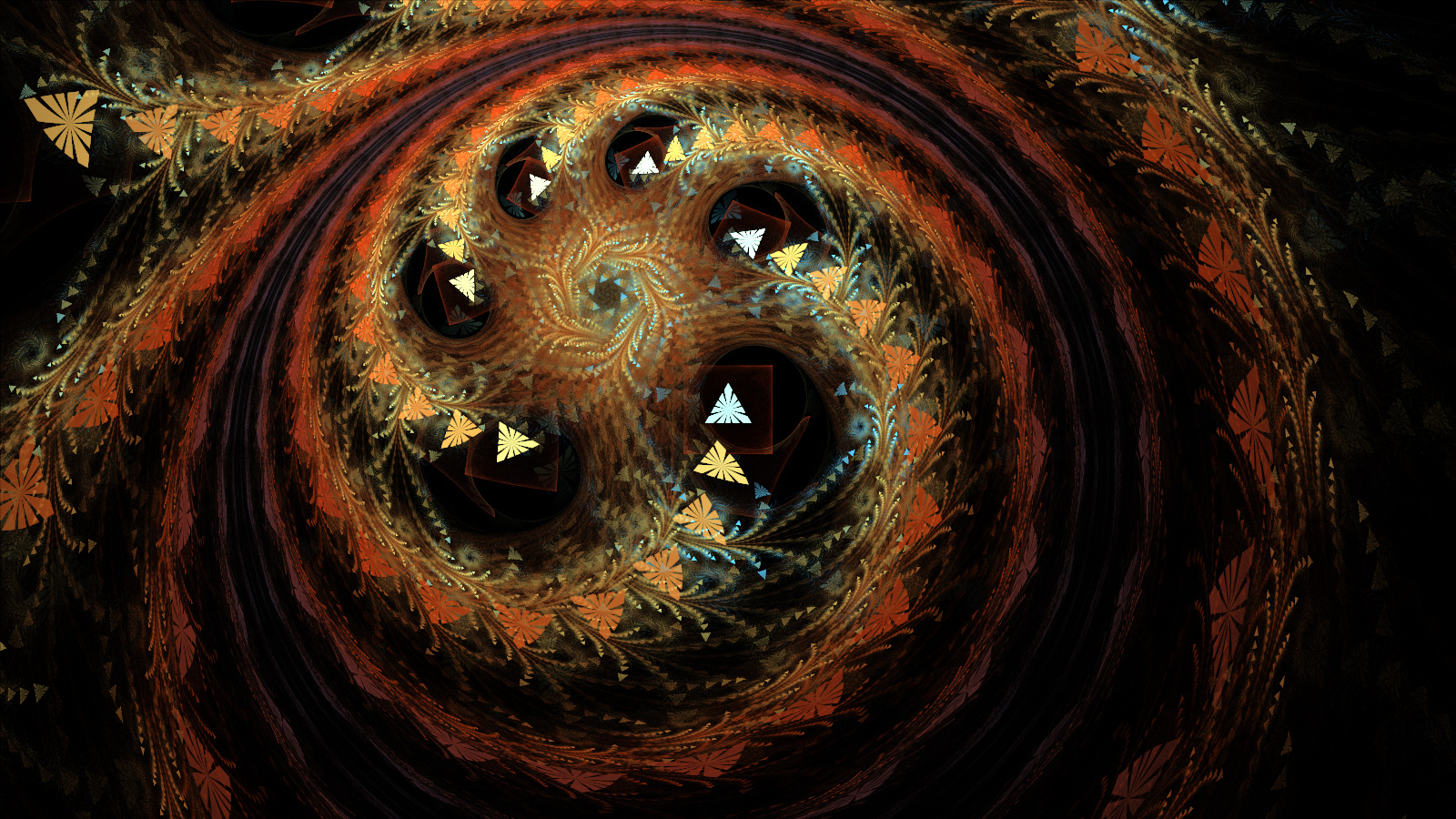The image showcases a vibrant, intricately designed spiral that appears as though it is formed from vines or branches. This swirling pattern is rich in color, featuring hues of orange, red, yellow, and hints of green and turquoise, giving it a textured appearance. As the spiral winds inward, the shapes transition into triangles, some of which resemble feathers or dried grass, contributing to the intricate detail of the design. Adding to the complexity, the center of the spiral holds a six-pointed star. The overall aesthetic resembles the cosmic beauty of a galaxy, with its swirling, floral-like structures and vivid color palette.